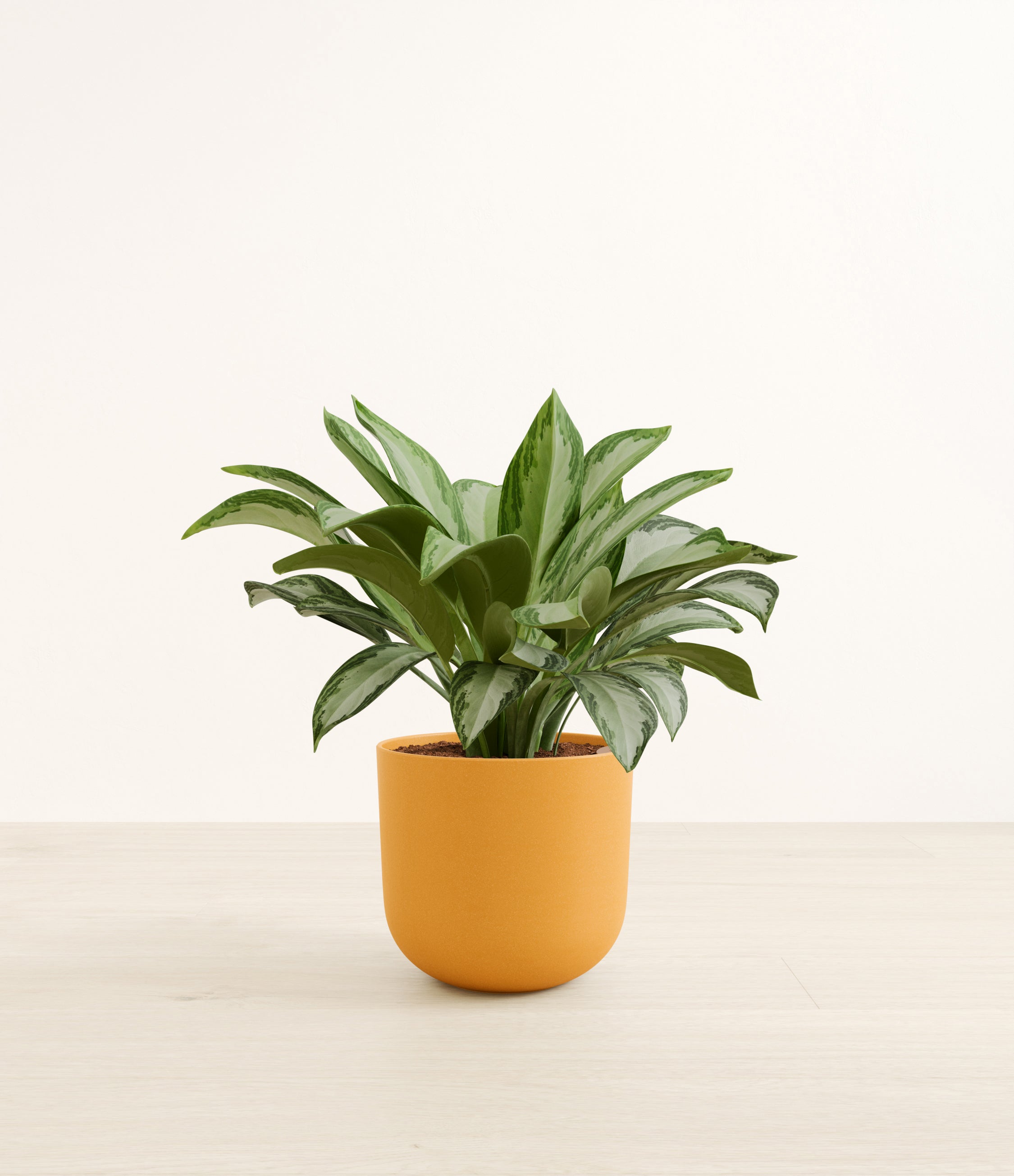The image features a vibrant green plant with numerous, spear-shaped leaves that radiate in various directions. The leaves are variegated, displaying dark green edges and lighter, almost silvery centers, with a distinct crease running down the length of each leaf. The plant sits in a plain, mustard-colored pot that has straight sides and a rounded base, lacking any drip tray or saucer. The pot is filled with visible brown soil. The setting includes a very pale, almost whitewashed wood surface, and a blank, tannish background that gradients slightly darker with subtle line patterns, but mostly appears white. The overall composition suggests a simple, yet healthy and flourishing plant arrangement.